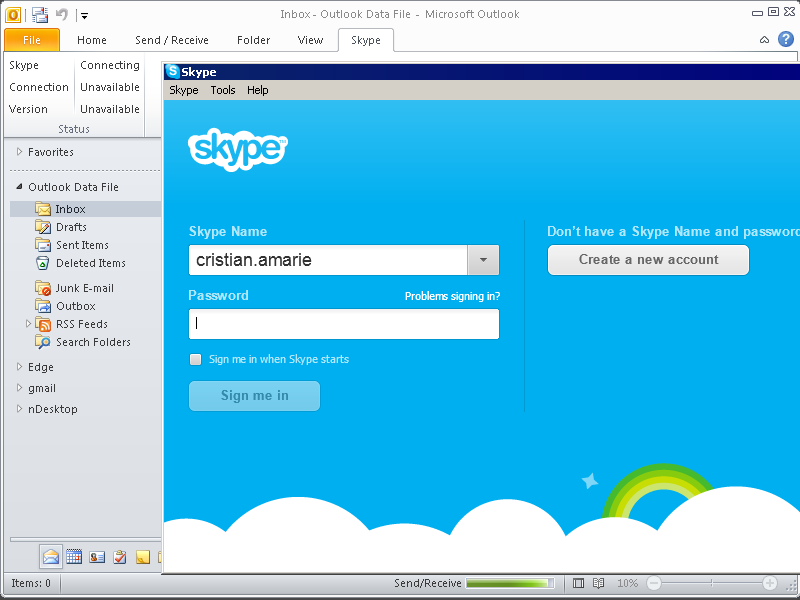Here is the cleaned-up and detailed caption for the image:

"The top left corner displays 'YOLO.' Adjacent to it are various icons and text labels such as 'Inbox,' 'Dash,' 'Outlook,' 'Datafile,' 'Dash,' 'Microsoft Log,' and 'MySQLX.' Beneath these, there are several tabs labeled 'File,' 'Home,' 'Census,' 'Read,' 'Folder,' 'View,' 'Skype,' 'Skype Connection,' 'Version,' 'Connecting and Available,' 'Remote Test,' and 'Columns.'

Under the 'Columns' section, the following categories are listed: 'Favorites,' 'Outlook,' 'Datafile,' 'Inbox,' 'Drafts,' 'Sent Items,' 'Deleted Items,' 'Junk Email,' 'Unboxed,' 'Artists,' 'Feeds,' 'Switch Folders,' 'Edge,' 'Gmail,' and 'Desktop.' 

There is an item labeled 'Item 0,' followed by 'Census,' and a green progress bar indicating '10%' completion. Next to the bar, there are icons for 'Minus' and 'Plus.'

At the bottom, options for 'Skype Tools,' 'Help,' and fields for 'Skype Name,' 'Skype Password,' and 'Skype Input' are repeated twice."

This detailed description highlights the different elements and text labels present in the image, providing a comprehensive overview.